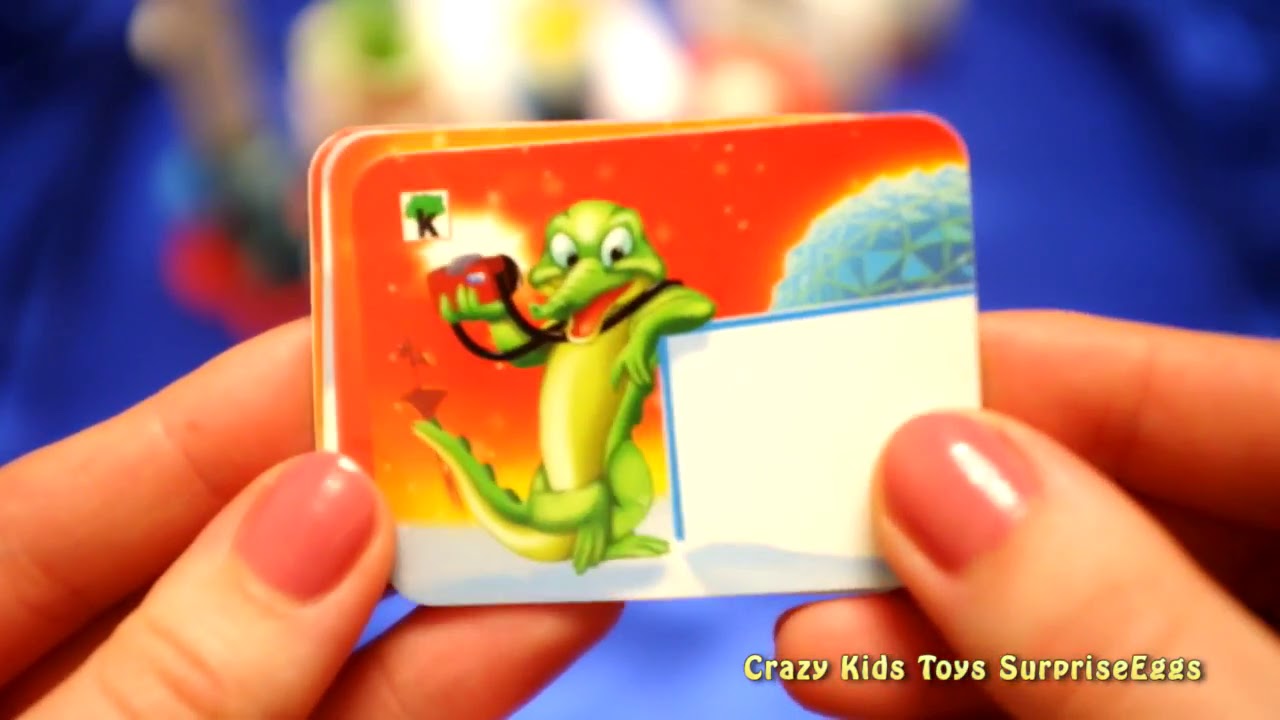The image depicts a person with pink nail polish on their thumbs, holding a rectangular card or toy square in the center of the frame. The card, prominently displayed against a blurry, largely royal blue background, shows an animated cartoon alligator standing upright and resting its arm on a white box outlined in blue. The alligator, which appears to be smiling, is holding a red object with a black strap around its neck. There is also an orange background featuring a white globe on the right-hand side of the card. Additionally, the top left corner of the card has a brown letter "K" with a green bush above it. In the bottom right corner of the overall image, there is text that reads "Crazy Kids Toys Surprise Eggs" in yellow letters, suggesting the image could be part of an advertisement or promotional material. The setting appears indoors, possibly in a child's room, with a focus on vibrant colors like blue, tan, red, light blue, green, yellow, orange, light green, pink, and white.